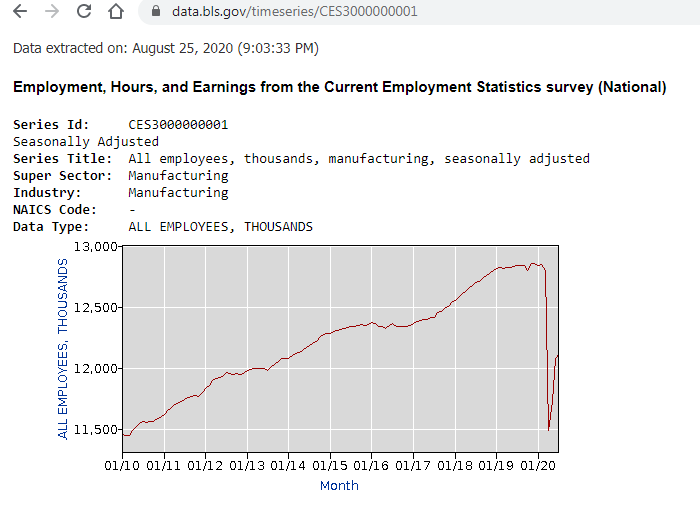The image depicts a detailed line graph with a white background. The graph itself is a gray rectangle featuring white grid lines and a red line illustrating data fluctuations. Above the graph is a comprehensive set of black text that provides contextual information extracted on August 25th, 2020, at 9:03:33 p.m. The title indicates that the data is from the Current Employment Statistics Survey National. The Series ID is CES3-0000-00-001, and the data is seasonally adjusted. Specifically, the series title is "All Employees, Thousands, Manufacturing, Seasonally Adjusted." The supersector and industry both fall under manufacturing, while the data type focuses on all employees measured in thousands. The URL provided is data.bls.gov/timeseries/CES30000001. 

Within the graph, the left vertical axis measures the number of employees in thousands, marked at intervals such as 11,500, 12,000, 12,500, and 13,000. The horizontal axis denotes the timeline, formatted as month and year, ranging from January 2010 (01/10) through to January 2020 (01/20). The red line starts from around 11,500 employees, peaks near 12,800, then sharply descends towards 12,000 by the 20th of January. The overall image looks like a screenshot from a web search engine, complete with navigation arrows and a URL input field, lending additional context to the data presentation.